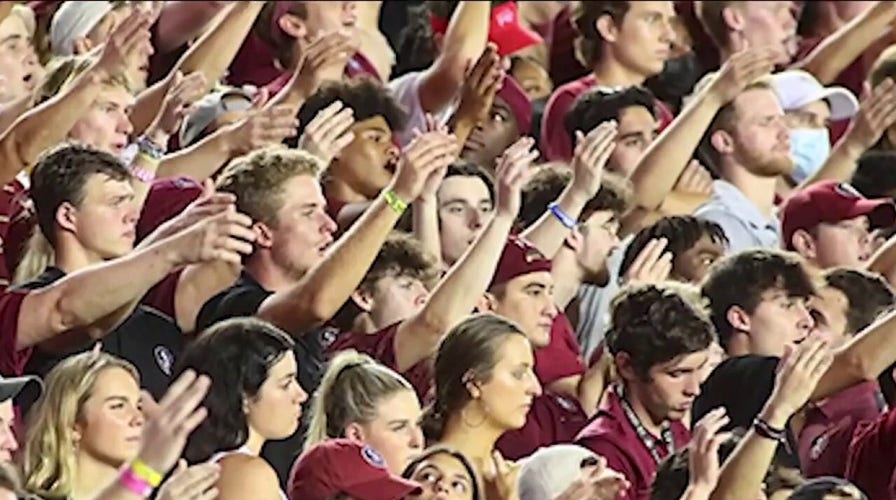The image depicts a close-up of a crowd, primarily composed of young men and a few women, likely college or high school students. They appear to be at a sports event, possibly supporting their team, given their absorbed and animated expressions. Most of the crowd is wearing maroon or burgundy attire, including shirts and hats with logos, indicative of school colors. The scene shows them with hands raised, possibly in celebration, clapping, or in a gesture of support or prayer, as they all direct their gaze to the right. Many individuals are adorned with wristbands and lanyards, adding to the event's uniformity and sense of unity. Despite the lively atmosphere, some faces appear distressed or bored, contrasting with the otherwise energetic display.